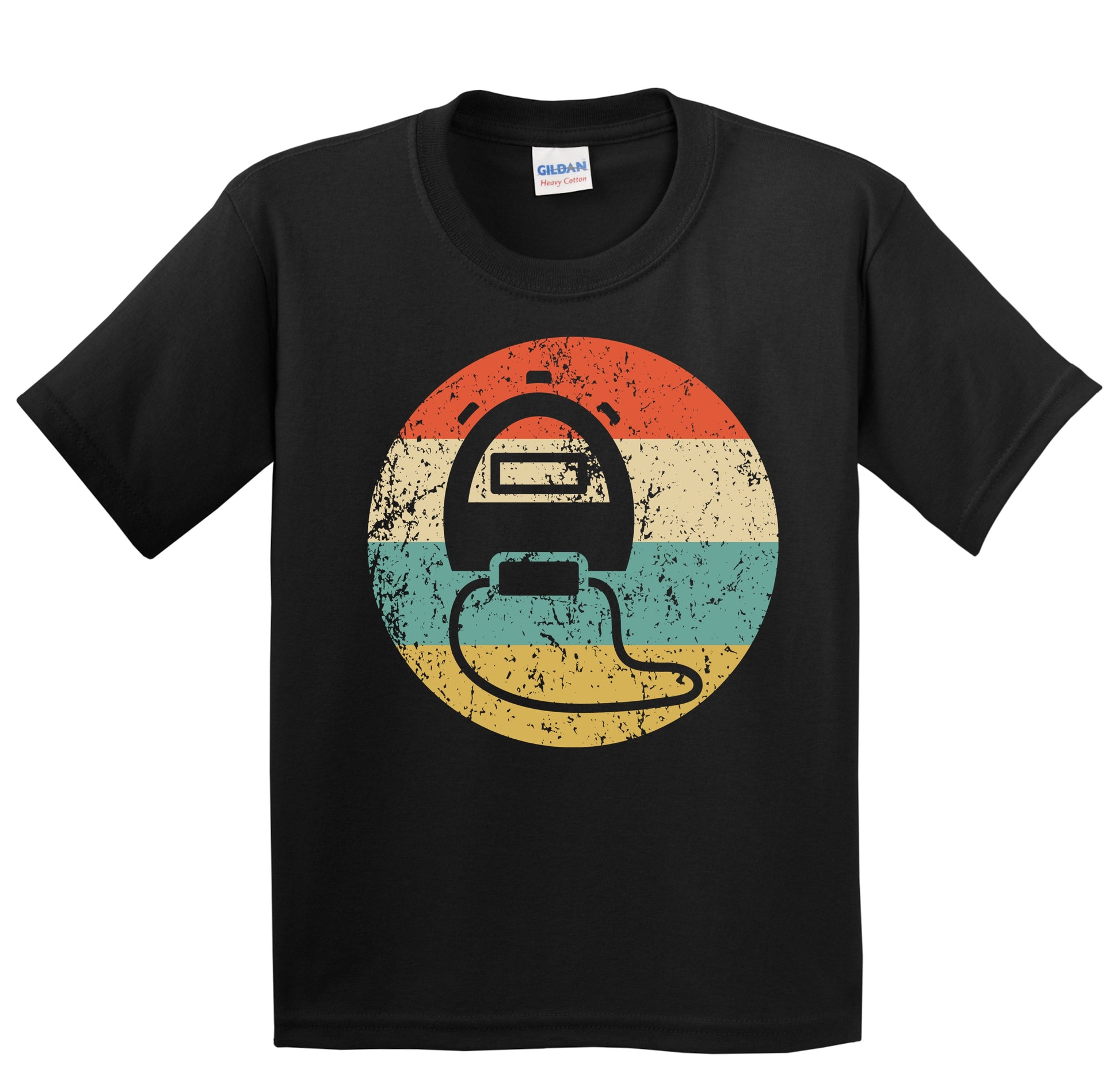This detailed image depicts a Gildan heavy cotton black t-shirt, likely unisex or men's, displayed against a completely white background suggestive of a product advertisement. The t-shirt features a standard design with a crew neck and short sleeves, accompanied by a small white tag on the back that has blue text reading "Gildan" and smaller, unreadable red text. Prominently centered on the t-shirt is a large, artistically styled circle logo showcasing a series of horizontal stripes in a retro color palette: red on top, followed by white, light blue, and yellow at the bottom. Superimposed on these stripes is a black silhouette resembling either a stopwatch, camera, helmet, or possibly an iron, adding to the abstract and intriguing nature of the design. A cord-like line extends from the base of this silhouette, while three additional lines appear above it. The overall look of the logo has a weathered effect, suggesting a vintage or worn-in aesthetic.